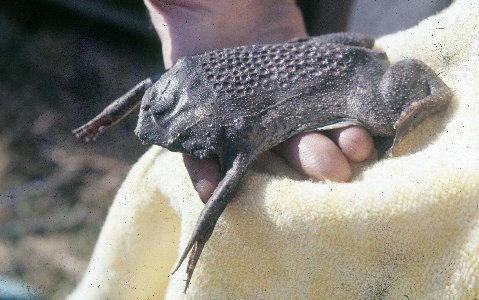In this grainy and horizontally aligned rectangular image, a hand, presumably belonging to a white individual, extends from the top of the frame holding what appears to be a lifeless frog. The frog, with its arms stretched straight out and legs curled behind, features small circular indentations on its back and exhibits a grayish-brown color with lighter spots near its face. There is ambiguity about the frog's authenticity, with some suggesting it might be metallic or artificial. In the blurry background, the left side contains brown sticks or branches, and there are patches of green and yellow grass. There is also some light blue in the lower left corner and a cloth material, possibly a white and yellow towel, under the frog in the top right corner. The frog itself is the focal point, with its inert form and distinctive pattern being most prominent.